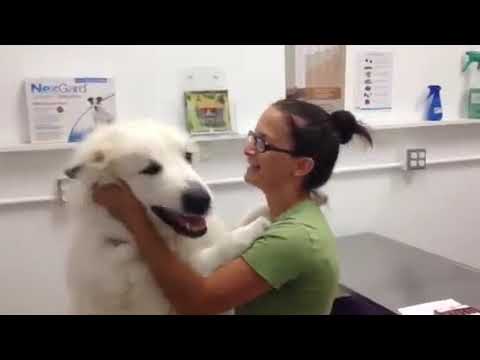In a brightly lit veterinarian's office, a white woman with brown hair, tied back in a bun or ponytail, is seen wearing glasses and a green shirt. She is warmly petting a large, white dog with a black nose and mouth, resembling a Great Pyrenees. The dog, standing on its hind legs with its paws on the woman's shoulder, appears content as it slightly opens its mouth, perhaps in a joyful pant. The background features a white wall adorned with various animal medicines, posters, and pamphlets, including Nexgard flea medicine. A gray table and a small blue spray bottle are also visible, providing additional context to the veterinary setting.